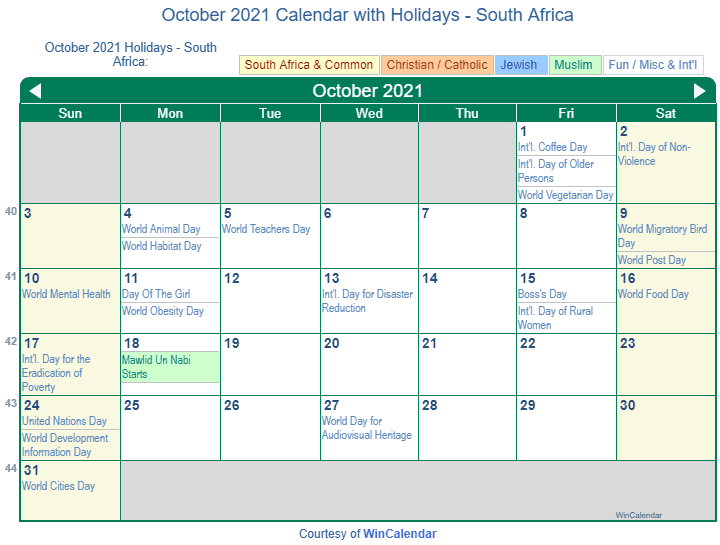Screenshot of October 2021 Calendar with Holidays - South Africa

This image is a detailed screenshot of an October 2021 calendar template, prominently titled "October 2021 Calendar with Holidays - South Africa" in blue font at the top. Directly below the title, the same text is repeated on the left side. On the right side, there is a color-coded key consisting of five different colored rectangles, each representing various event categories: "South Africa," "Christian Catholic," "Jewish," "Muslim," and "Fun and Miscellaneous and International."

The calendar itself is bordered in green, with a green banner at the top displaying "October 2021" flanked by navigation arrows on both sides. The days of the week are clearly labeled at the top of the calendar grid. Days not belonging to October are shaded in gray, while weekends are highlighted in yellow. The weekdays are presented against a white background.

The calendar features a mix of blank squares, indicating no events, and squares containing lists of events in blue text. Notably, October 18th is marked by a green rectangle, indicating a Muslim holiday. Other highlighted or listed events fall under the "Fun and Miscellaneous" category, which are shown in blue or against a white background without specific highlighting.